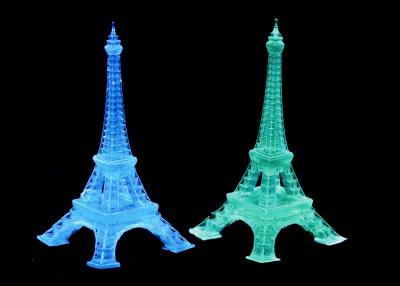The image displays a striking contrast of two glowing Eiffel Tower-like structures set against a deep, solid black background. The rectangular image, which is slightly wider than it is tall, features these towers side by side. Both towers, depicted in a vibrant, neon-like glow, appear to be illuminated as if they can glow in the dark. The tower on the left is bathed in a radiant blue light, while the one on the right glows in a vivid green hue. Each structure captures the iconic form of the Eiffel Tower, though the green tower leans slightly more to the right, giving a subtle variation in angle. The black background accentuates the luminescence of the towers, making them the exclusive focal points of the image, with no other objects, words, or letters present. The clarity of the image ensures the distinct lighting and colors of the towers stand out brilliantly against the dark backdrop.